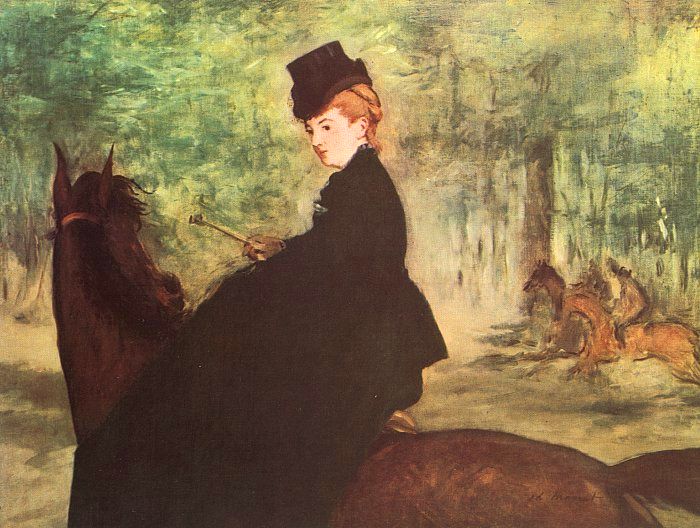The painting depicts an outdoor scene set in a forest, with a woman riding side saddle on a large brown horse. The foreground is dominated by the woman, who has fair skin, reddish-brown hair pulled back in a bun, and brown eyes. She wears a black riding gown that covers her from neck to ankles, along with a hat decorated with lace and a black band. Her right hand, clad in a brown glove, holds a riding crop. The horse’s head is turned toward the other horses, showing the halter strap across its head. The background features a forest with trees characterized by green leaves and brown trunks, rendered in broad strokes that suggest rather than detail the foliage. Blurry outlines of two additional horses with riders can be seen to the right, partially obscured by the forest setting, contributing to the depth of the scene. The overall palette of the painting includes greens, browns, and touches of white and tan. The woman’s gaze is directed slightly downward and to her left, creating a sense of contemplation and movement within the tranquil woodland environment.